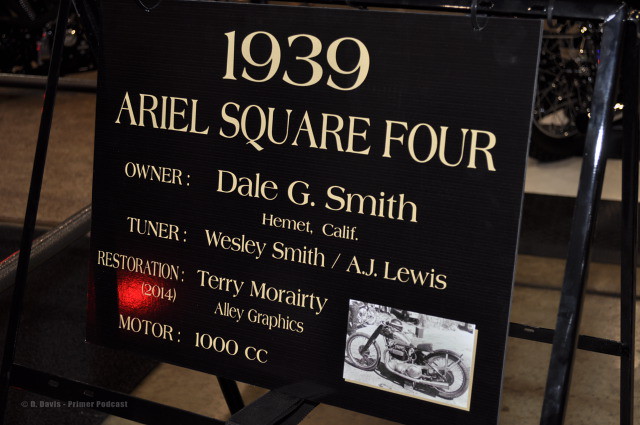The image depicts a detailed informational plaque mounted on a black metal frame, likely in an interior setting such as a museum or car show with a concrete floor. The central focus of the image is this square black plaque, which features text in a light yellowish color. The prominent text at the top reads "1939 Ariel Square 4" in large font. Below, it specifies: "Owner: Dale G. Smith, Hemet, California; Tuner: Wesley Smith / AJ Lewis; Restoration: Terry Moriarty, 2014; LE Graphics; Motor: 1000 CC." In the bottom right corner of the plaque, there's a small black-and-white image of a motorcycle. In the background, part of the motorcycle displayed on a white platform can be slightly seen. The plaque is attached to the metal frame using zip ties.